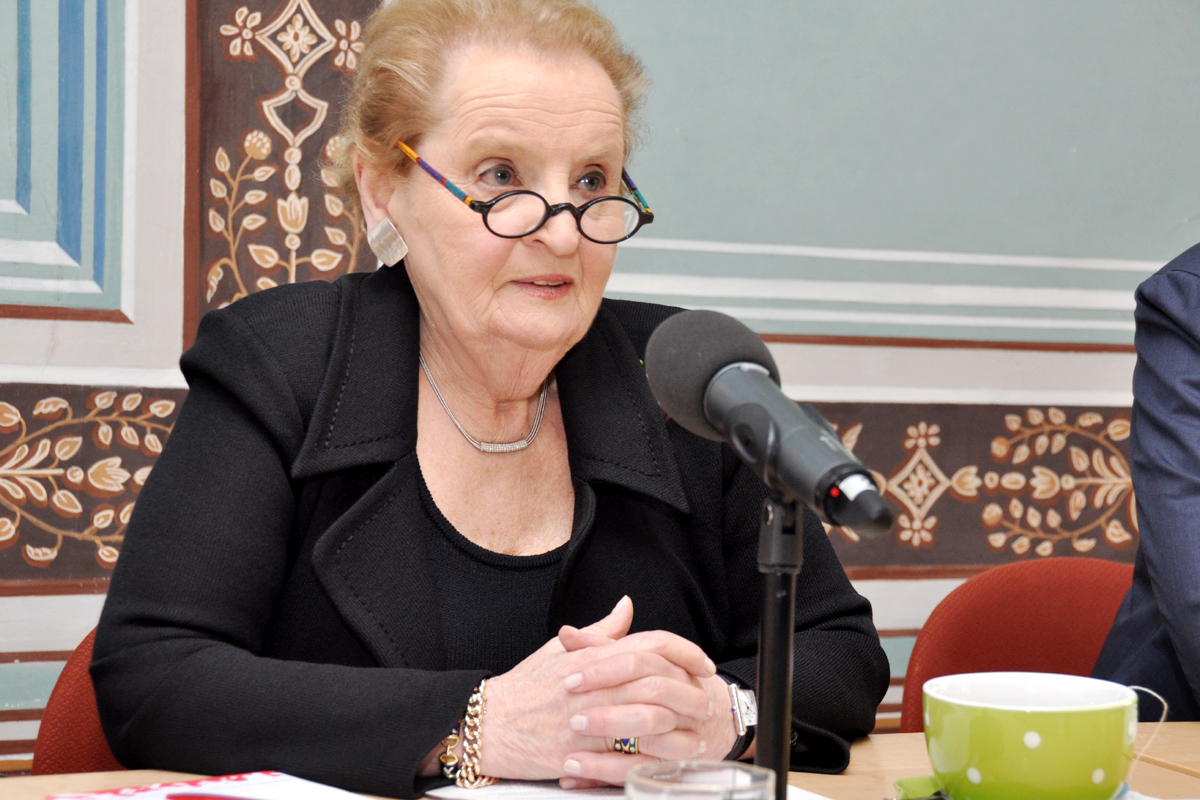In this indoor setting, the image captures a scene centered around an older woman, who closely resembles Madeleine Albright, seated at a wooden table. The table holds various objects, including papers and a green teacup. Seated directly in front of a microphone, the woman is engaged in speaking, her hands folded. Her attire includes a black suit jacket and a matching blouse, accessorized with colorful, bold-framed glasses, large diamond-shaped earrings, a silver necklace, bracelets, and a ring. Her light orange hair is pulled back, possibly to mask a thinning spot, and she's perched her glasses low on her nose, peering over them as she addresses her audience.

The scene is visually rich with colors like light blue, blue, white, maroon, brown, orange, light green, and gold. Surrounding the table are red chairs, with another individual visible on her left, wearing a navy suit jacket. The background features a wall adorned with floral brown wallpaper, accented with sections of blue, suggesting the setting is a formal meeting or conference room. The woman, centrally positioned, commands attention with her poised yet attentive demeanor, making this a detailed and intimate portrayal of a significant event or discussion.